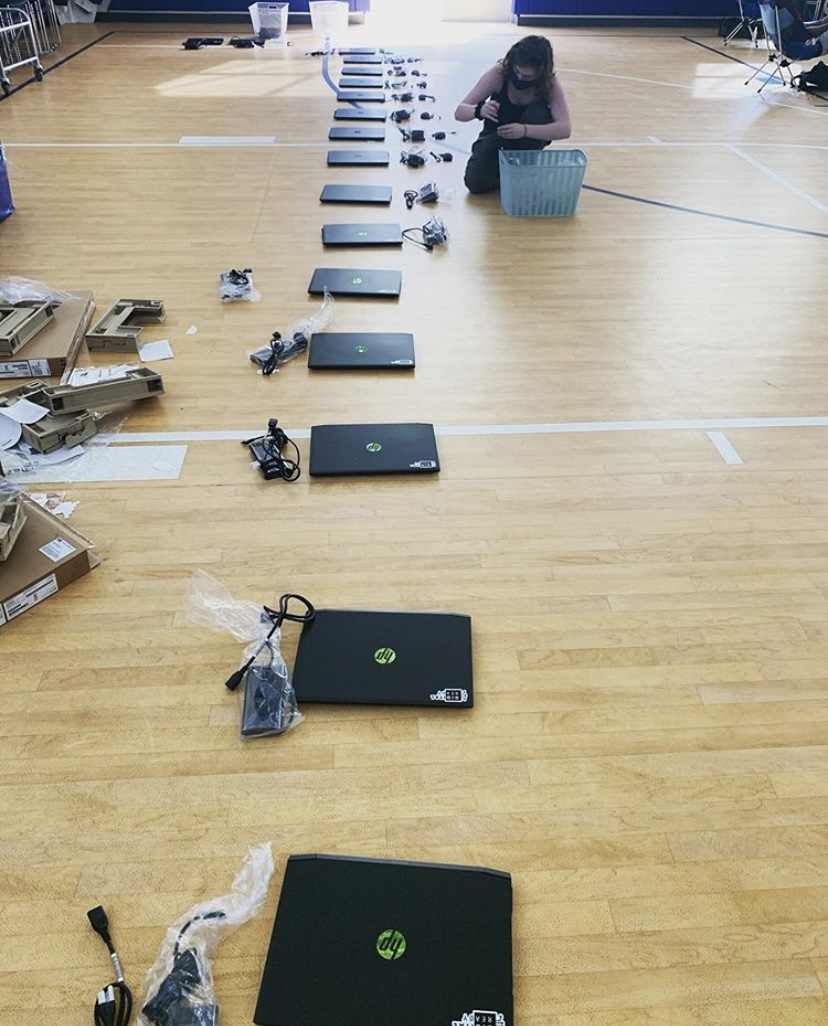This color photograph captures a scene within what appears to be a gymnasium, indicated by the large wooden floor with visible basketball court markings, including intersecting horizontal lines and a rounded boundary at the top. Arranged in a long vertical line across the floor are numerous black HP laptops, each adorned with a green sticker bearing black lettering. Many of these laptops have power cords emerging from the left side, with the first few cords encased in clear plastic bags. The further back the laptops are, the more the cords seem to exit from the right-hand side, and these cords are not bagged.

At the upper portion of the image, a woman with dark hair wearing black is seen kneeling beside the laptops, examining a blue, almost translucent box in front of her. Nearby, there's additional equipment and opened beige-brown laptop packaging scattered on the left side, suggestive of recent unboxing. A white trolley is also visible in the upper left corner, while the upper right corner hints at a blue object that might be a chair. The environment is illuminated by a light source from above, possibly near a window or door, with a dark blue wall in the background. Each laptop bears a blue and white symbol at the bottom right corner, reinforcing the setup's orderly yet preparatory nature.